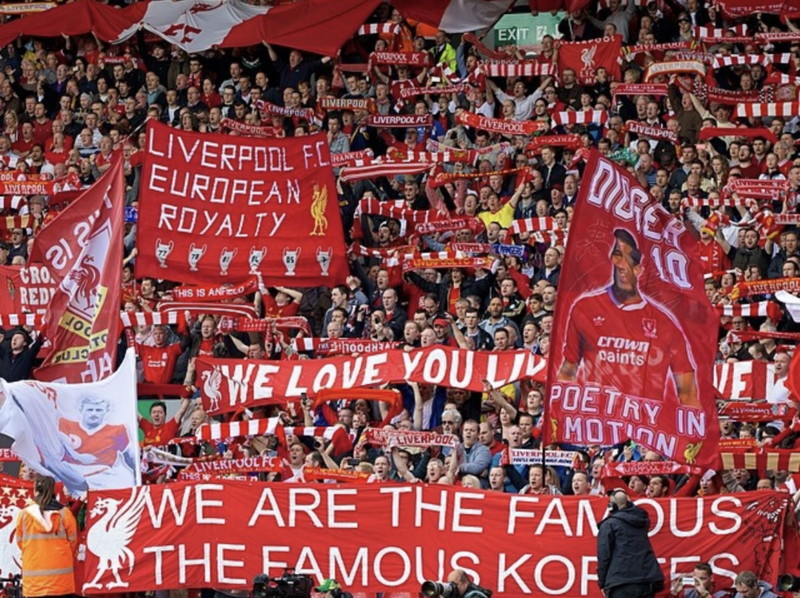The image depicts a packed stadium filled with Liverpool FC fans, emblazoned in the team's signature red and white colors. The stadium is brimming with jubilant supporters holding up various banners and signs. A prominent banner near the top reads "Liverpool FC European Royalty," accompanied by the club's iconic griffin logo scattered throughout the scene. Another significant banner showcases a player, numbered 10, wearing a red jersey with "Crown Paints," and the phrase "Digger 10 Poetry in Motion." At the bottom, a long horizontal banner boldly states "We are the famous, the famous copies," flanked by white and red phoenix insignias. Security personnel in orange jackets and a photographer with a black jacket and headphones are also visible. The crowd, predominantly composed of men clad in red and white scarves and sequins, is animated, cheering, and waving their hands, creating an electrifying atmosphere that suggests their team is performing well.